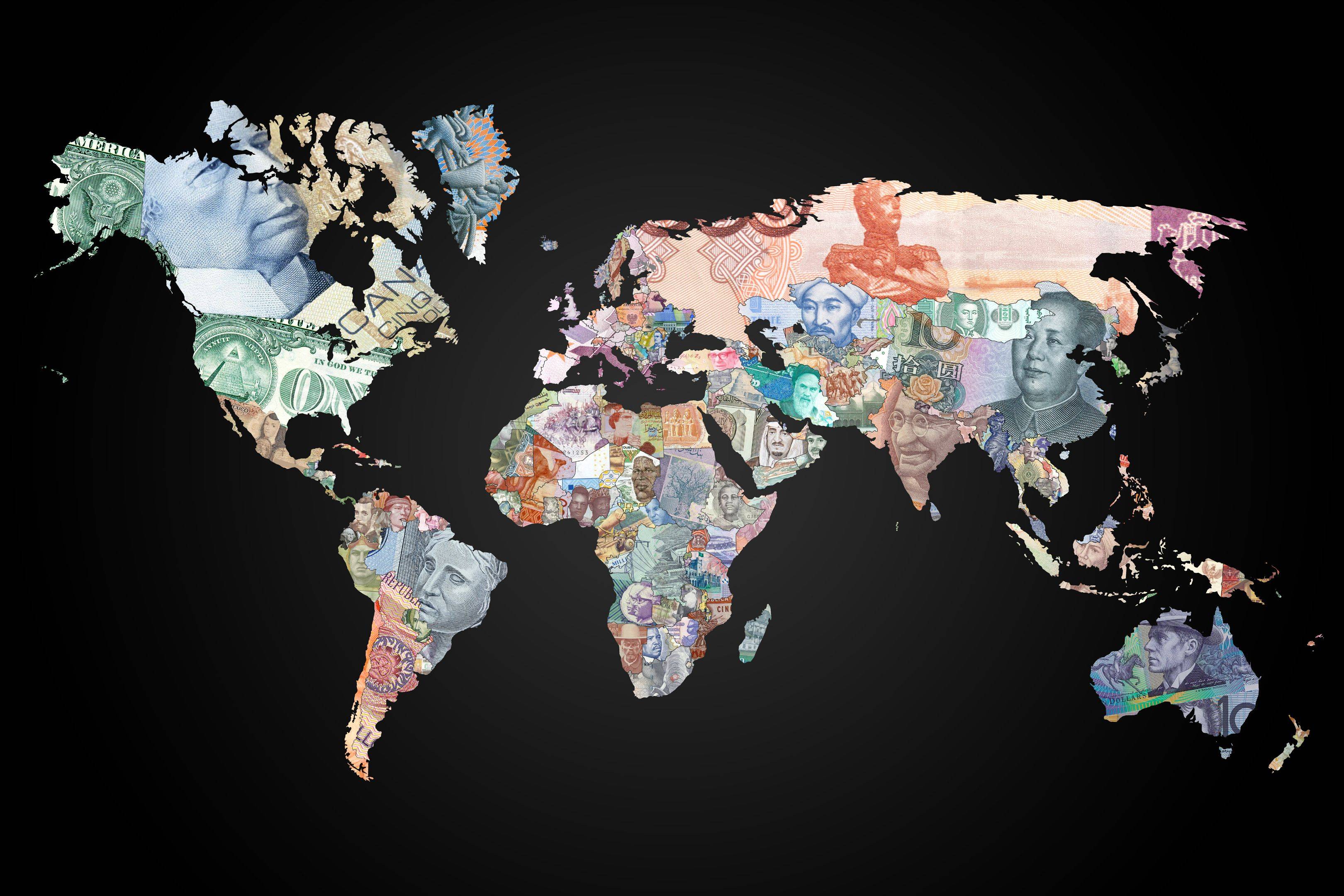In this rectangular image, the entire world map is creatively reimagined against a stark, solid black background. Unlike a typical map displaying country borders and names, this artistic rendition features vivid, colorful illustrations of various world leaders superimposed over the continents they represent. The artwork includes noticeable depictions of Middle Eastern leaders, figures adorned in traditional Asian attire, and what appears to be a prominent United States president. The contrast between the solid black backdrop and the vibrant, detailed illustrations of the leaders makes the image striking and captivating. The black background, devoid of any shading, ensures that the colorful and intricate illustrations stand out prominently, offering a unique, symbolic portrayal of global leadership.